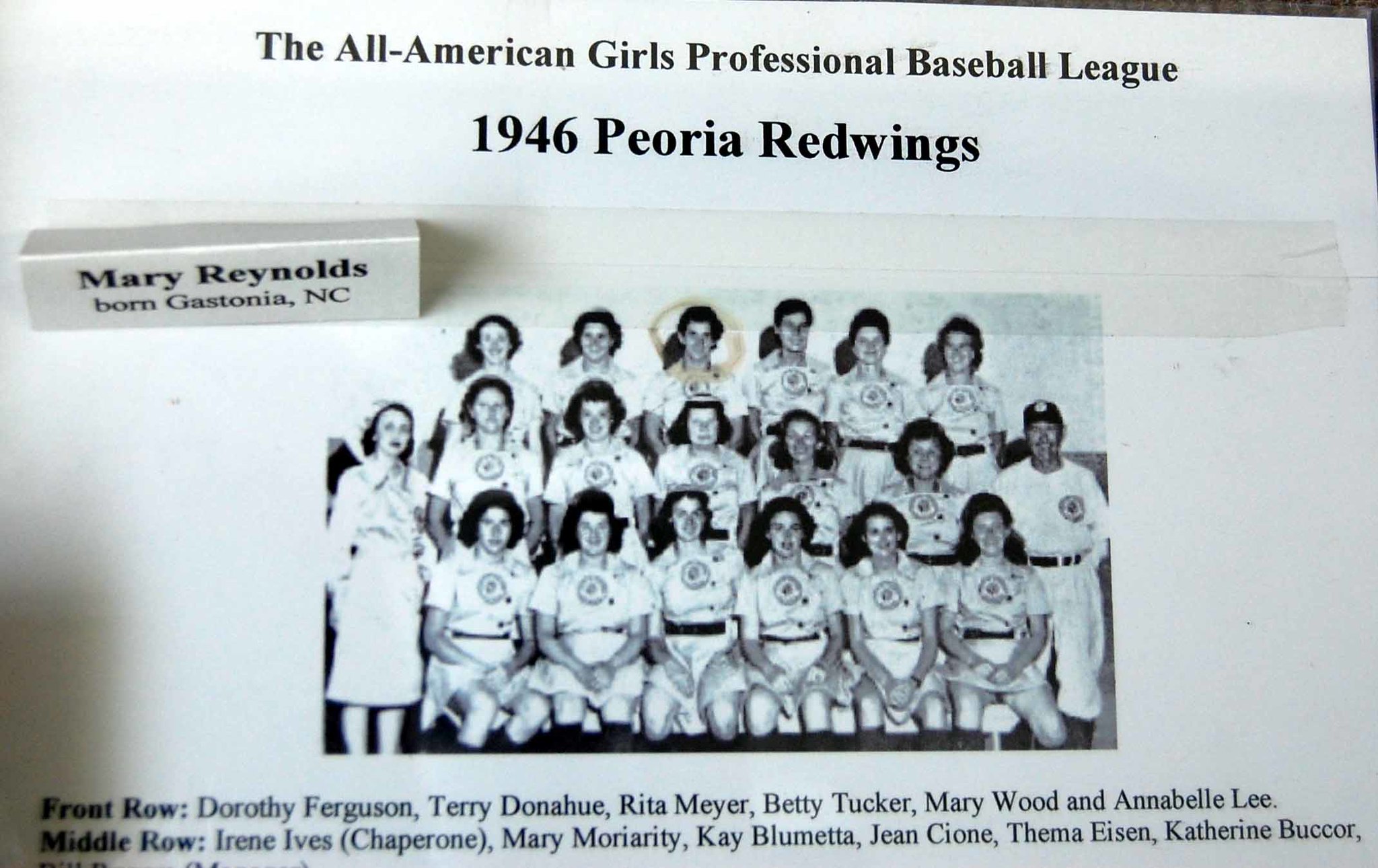A black-and-white photograph captures the 1946 Peoria Red Wings of the All-American Girls Professional Baseball League. The image shows a grainy, historical moment with the team arranged in three rows. The front row features Dorothy Ferguson, Terry Donahue, Rita Meyer, Betty Tucker, Mary Wood, and Annabelle Lee. In the middle row, Irene Ives (Chaperone), Mary Moriarty, Kay Blumetta, Jean Sion, Thema Eisen, and Katherine Begore are pictured. Though finer details are hard to discern due to the photo's age, one girl's head is circled. The back row includes two men positioned in the center; one appears to be a coach on the far right, and a nurse stands on the far left. A piece of folded paper taped above the photo identifies Mary Reynolds, born in Gastonia, North Carolina. The nostalgic tone of the image is underscored by its grainy quality and visible tape, capturing a cherished memory from the league's history.